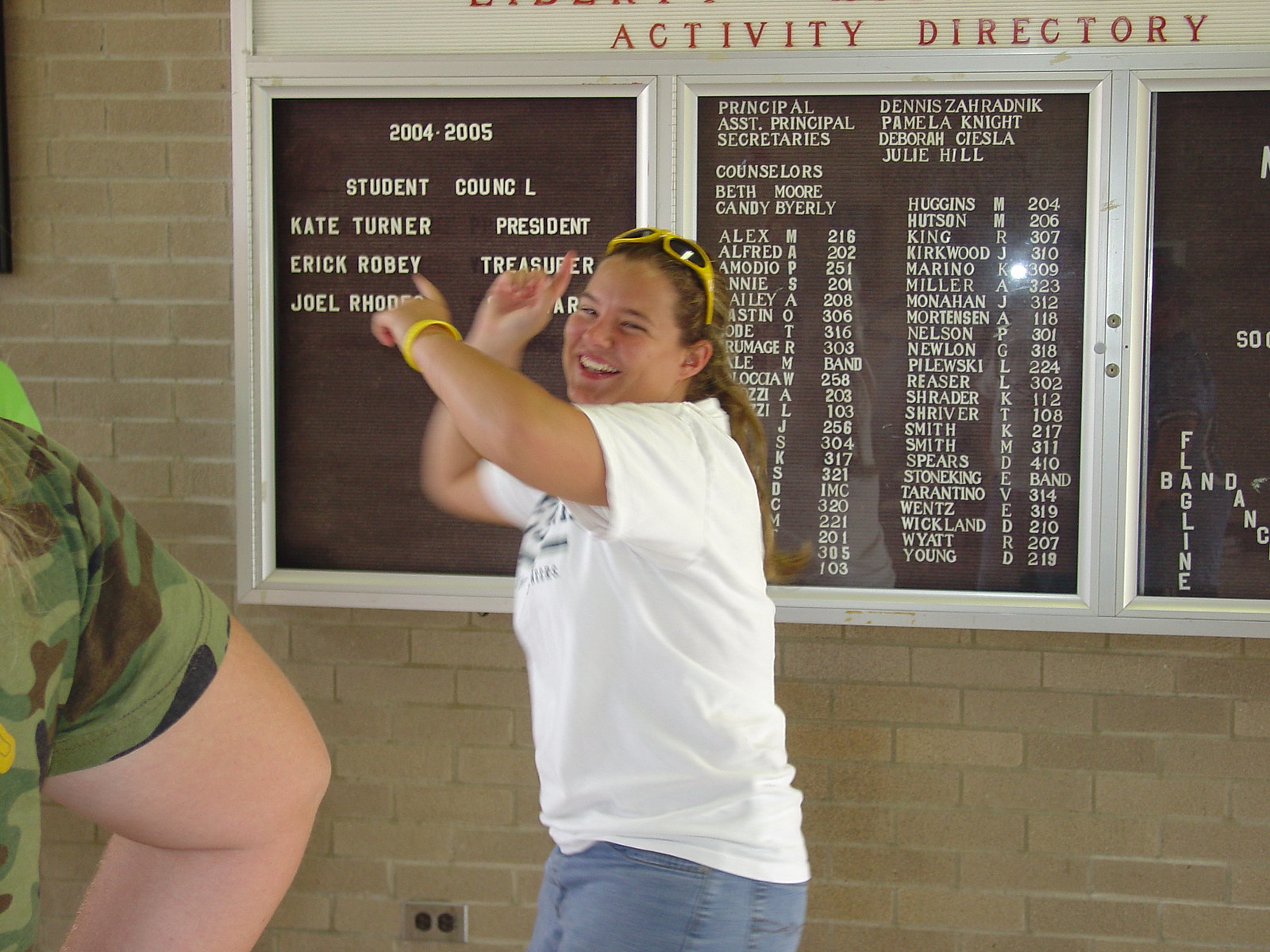A woman stands next to a reflective glass notice board divided into three black panels set in metal frames. She wears yellow sunglasses perched on her head, a white t-shirt, and jeans, and has a yellow wristband on her left wrist. Her hands are raised, partially obscuring some text on the left panel, and she is smiling and laughing. The board reads "2004-2005 Student Council" on the left panel, listing Kate Turner as President, Eric Roby as Treasurer, and partially showing the name Joel Rhodes. The middle panel identifies the school administration, which includes Principal Dennis Zadranik, Assistant Principal Pamela Knight, Secretaries Deborah Ciesla and Julie Hill, and Counselors Beth Moore and Candy Byerly. The right panel lists multiple columns of names and apparent room numbers.